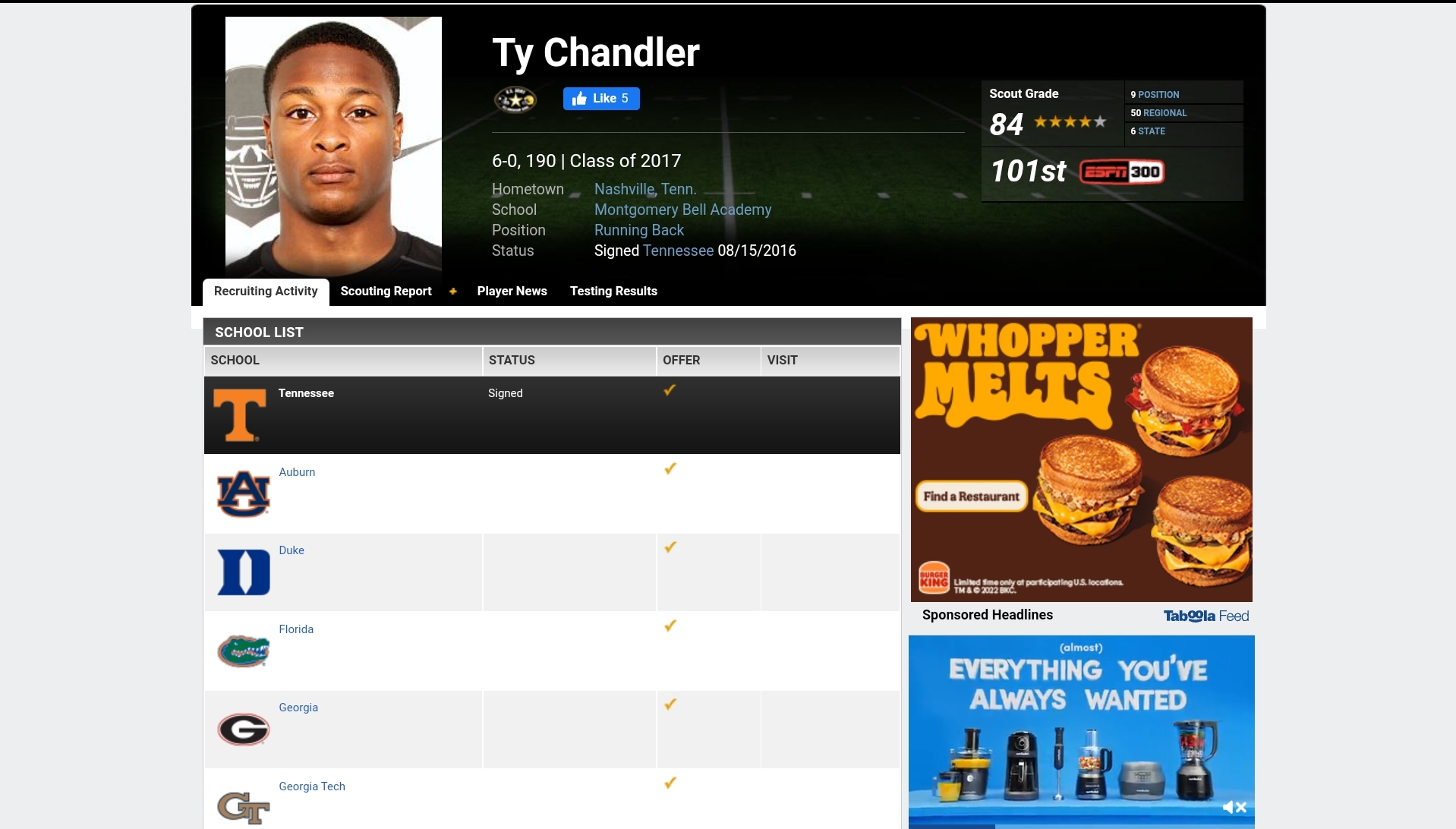The image appears to be taken from an ESPN website and showcases an in-depth scouting report for a high school athlete. At the top of the image, there is a picture of an African-American young man, identified as Ty Chandler, with helmet emblems visible in the background. Below his photo, the text prominently reads "Scouting Report" and provides detailed information about his recruiting activity.

The left column lists various schools that have shown interest in Ty Chandler, including Tennessee, Auburn, Duke, Florida, Georgia, and Georgia Tech. Adjacent to this column is a "Status" section, which is mostly unchecked for "signed" status, indicating he has not signed with any of these schools. In contrast, the "offer" column has every box checked, signifying that he has received scholarship offers from all the listed colleges. The "visit" column has no check marks, implying he has not made official visits to these schools yet.

At the top of the report, additional details about Ty Chandler are provided: he is from Nashville, Tennessee, and attends Montgomery Bell Academy. His position is running back, and he signed with the University of Tennessee on August 15, 2016. The right side of the image contains several advertisements, including one for Burger King, and some sponsored headlines.